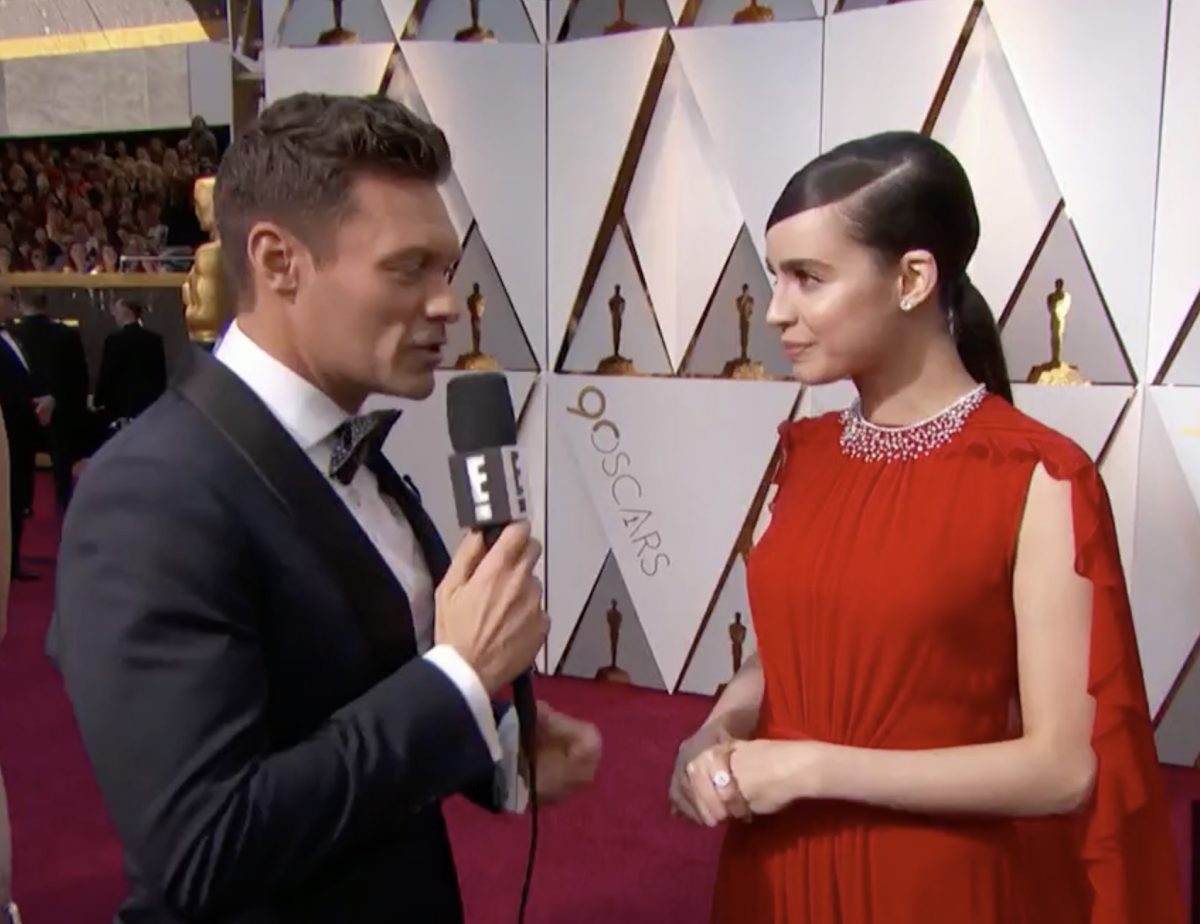This photograph captures an interview on the red carpet at the 90th Oscars, featuring Ryan Seacrest and Emilia Clarke. Ryan Seacrest, standing on the left side of the image, is sporting a black tuxedo with a white shirt and holds an E-network-branded microphone in his right hand. He is mid-question, facing Emilia Clarke, who is known for her role as Daenerys in Game of Thrones. Clarke is dressed in a sleeveless red gown, complementing her diamond necklace adorned with dangling jewels. Her dark brown hair is elegantly slicked back into a ponytail and parted on the left. She stands with her hands clasped at her waist, displaying a few rings. The red carpet beneath them appears slightly maroon or purple. The backdrop behind them features a wall with triangular patterns and silhouettes of the Oscar statues, along with the "90 Oscars" logo written in gold. Additional figures, dressed in black tuxedos, and a crowd of onlookers are visible in the background, highlighting the bustling atmosphere of the event.